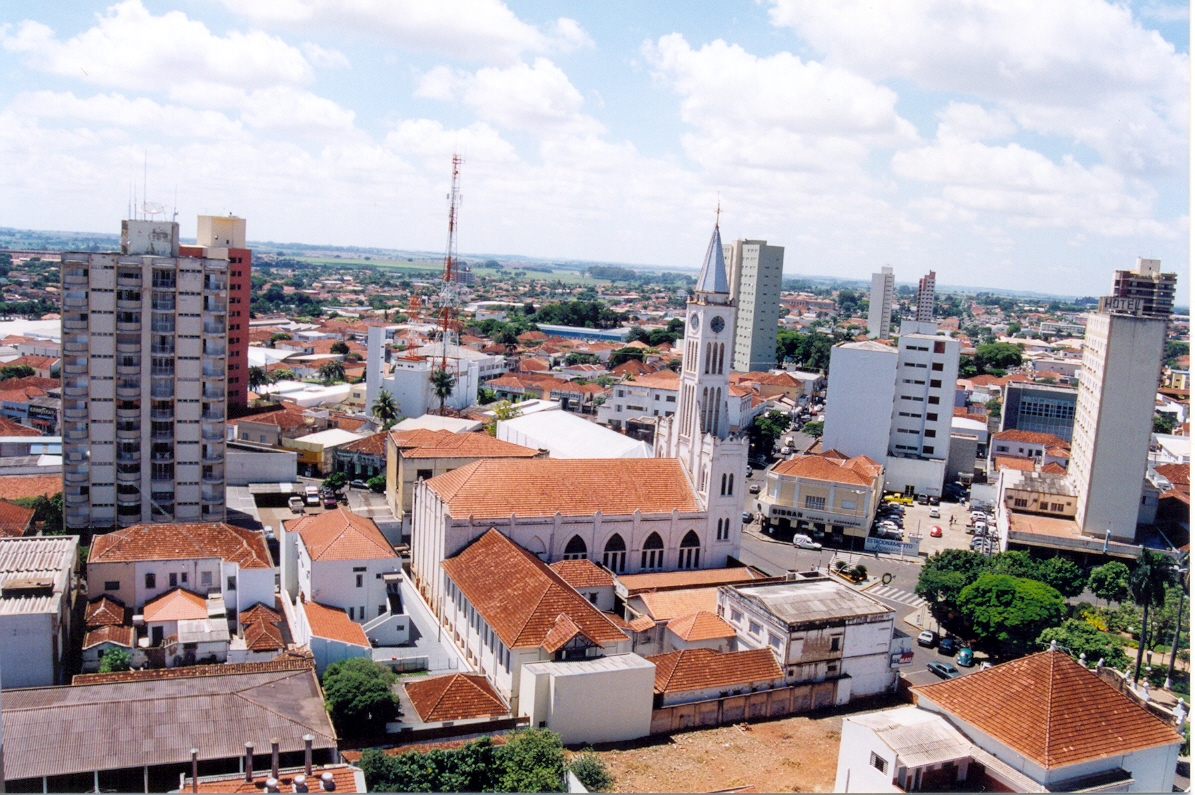The photograph captures a vibrant cityscape under a blue sky dotted with fluffy white clouds. In the forefront, numerous buildings with brownish-orange tiled roofs of various shapes and sizes create a picturesque, somewhat older city scene. To the left, two tall, modern hotels with small balconies stand out prominently. On the right, a couple of similarly tall tower-type hotels can be seen. Dominating the middle of the image is a large church-like structure with a very tall, light blue steeple, though it could also be a civic building given its clock. The town below is interspersed with green foliage and trees, creating a scattered pattern of greenery amidst the buildings. A noticeable feature is the red and white radio tower near the center, adding an industrial touch. On the far left of the scene, an intersection of streets forms an angle, bordered by a green parkway. The background extends to a green pasture, melding the urban and rural landscapes together beautifully.